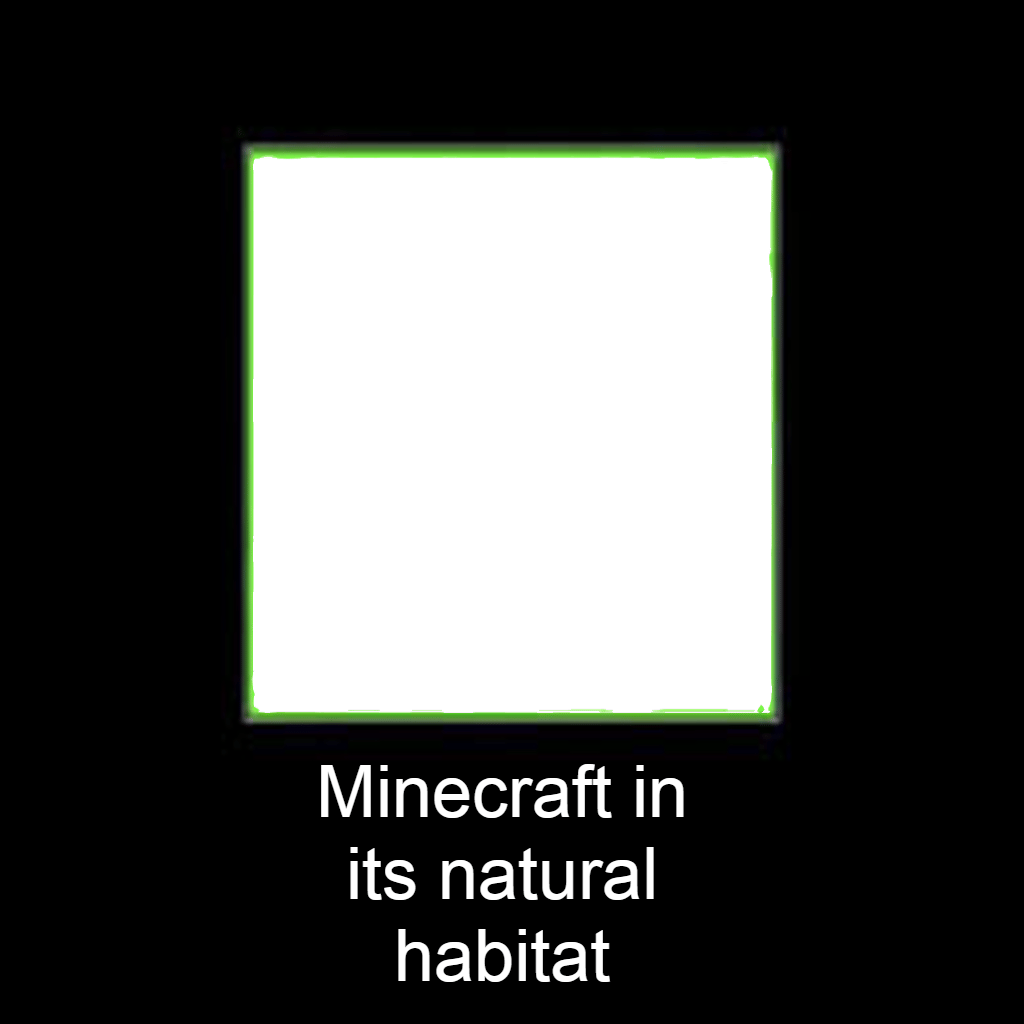The image features a minimalist design with a matte black background. In the center, there is a large white square, bordered by a very thin, faint green line that resembles watercolor. Underneath the white square, in moderately large, simple white text, it reads, "Minecraft in its natural habitat." This simple yet clever meme implies that Minecraft, the popular video game created by Mojang and developed by Notch, is fundamentally a series of squares or cubes, humorously represented by the plain white square with a green border.